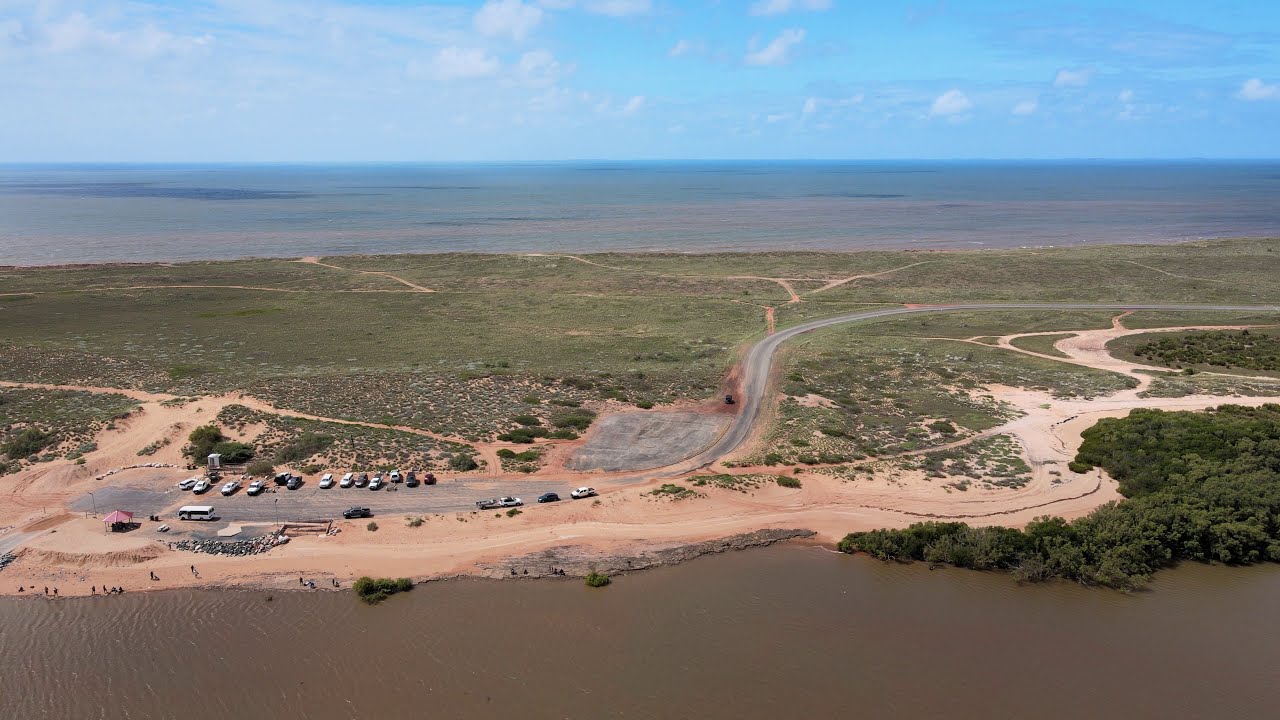This aerial image, possibly taken by a drone or from a high altitude, captures a sprawling outdoor scene in the middle of the day. At the bottom of the image, there is murky brown water, likely a river, with trees growing out of it at the bottom right. A dirt shoreline extends from the water, leading up to an asphalt road that curves and features about 15 parked vehicles, including a large bus. Some cars appear to be pulling boat trailers, and approximately 12 people can be seen fishing along the shore. The asphalt road is flanked by multiple dirt paths on both sides, which meander through a vast field of green grass and sparse vegetation. The horizon is dotted with patches of tan and red from dirt and buildings, adding a sense of depth to the landscape. Toward the top of the image, the blue sky is filled with clouds, and there is a hazy, distant object that might be a plane. The blended colors of brown, green, tan, red, orange, blue, gray, and white, along with the open layout, encapsulate the essence of nature and human activity coexisting in a serene outdoor setting.